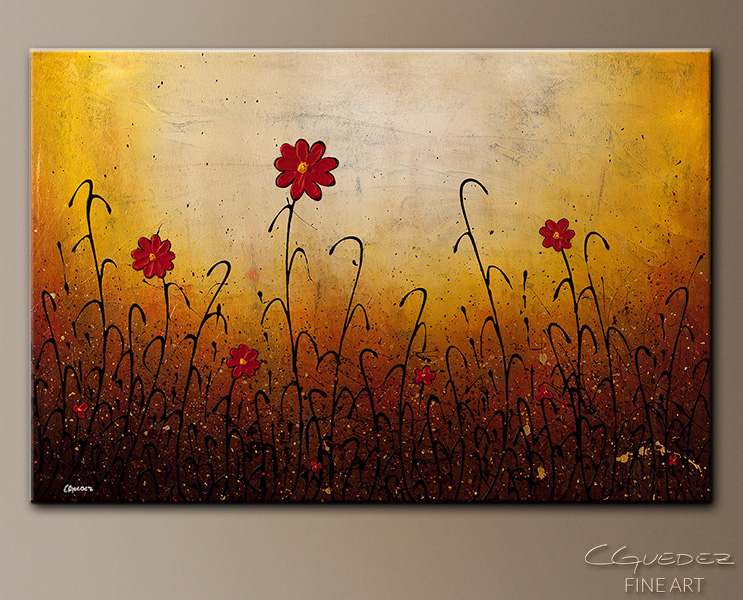This image showcases a photograph of an oil painting by C. Gudez, prominently signed in white cursive text in the lower left corner, with "Fine Art" inscribed on the right side. The painting, rendered in an illustrative style on a canvas set against a beige brown background, depicts a vibrant field of flowers. Eight red flowers, each with rounded petals surrounding orange or gold centers, dominate the scene. The flowers' stems are drawn with artistic, black, J-shaped curves and are surrounded by plant silhouettes featuring curved, hook-like leaves. The larger flowers are situated in a beige-yellow accented area near the top of the painting, while smaller flowers appear at the base and the corners. The background transitions from golden yellow at the top to dark brown at the bottom, effectively framing the blooming flowers.